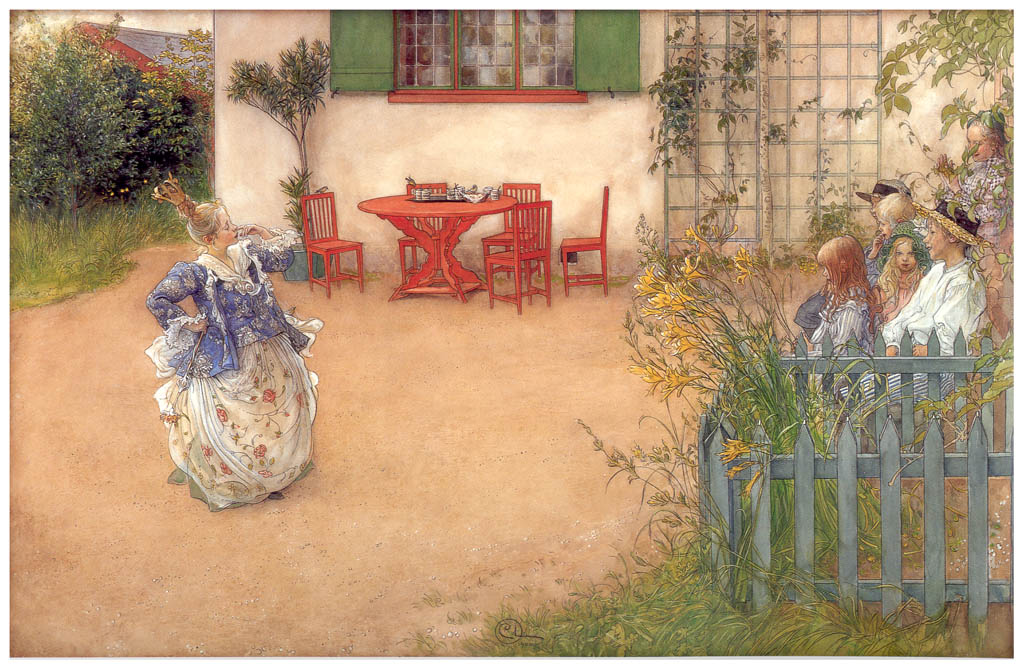The painting depicts a charming outdoor scene with a white building in the background, adorned with green-shuttered windows and a trellis covered in vines. In front of the building, there is a red table surrounded by four to five empty orange-red chairs, with a few cups and a potted plant on the table. On the left side of the composition, a woman dressed in a Victorian-style outfit stands on a dirt or concrete surface. Her attire includes a flowy white dress decorated with reddish flowers and a purple or blue top. She has her hair styled in a bun and appears to be holding one finger up to her nose, possibly wearing a crown. 

To the right side of the painting, a group of people—primarily young girls along with a couple of children, some wearing straw hats—sit behind a blue picket fence, attentively watching the woman. Behind them, tall yellow flowers, likely daffodils, grow inside the fenced area. The background also features another building to the left and some visible trees and grass, completing this picturesque setting.